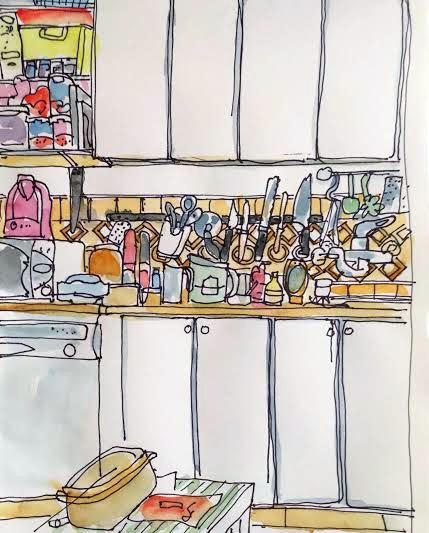This image is a detailed drawing of a cozy kitchen. The kitchen itself predominantly features a palette of white and beige, with warm yellow accents adding a cozy feel to the scene.

In the foreground, there is a prominently drawn kitchen countertop. On this countertop, you can see a pot along with a pot holder beside it. The countertop is bustling with activity and various items: there are several bottles and a pitcher placed in an orderly fashion.

Moving back, the focal point of the image is a well-detailed dishwasher. The artist has taken care to include the smaller elements like the knob and the buttons, which indicate the different wash settings. Below the dishwasher, there are kitchen cabinets featuring two circular knobs.

On the counter above the dishwasher, there is a variety of cookware hanging from a rack. This includes several knives, spoons, spatulas, and even a pizza cutter. The rack is drawn to suggest how kitchen tools are within easy reach.

To the far left of the drawing, a microwave is illustrated, complete with a knob. It appears to have a coffee pot or some kind of pot on top of it. Above the microwave, another row of cabinets is depicted, most of them closed except for one, which is open to show some storage containers inside.

This detailed sketch captures the essence of a functional and inviting kitchen, with various utensils and appliances meticulously illustrated to give a sense of everyday life in the space.